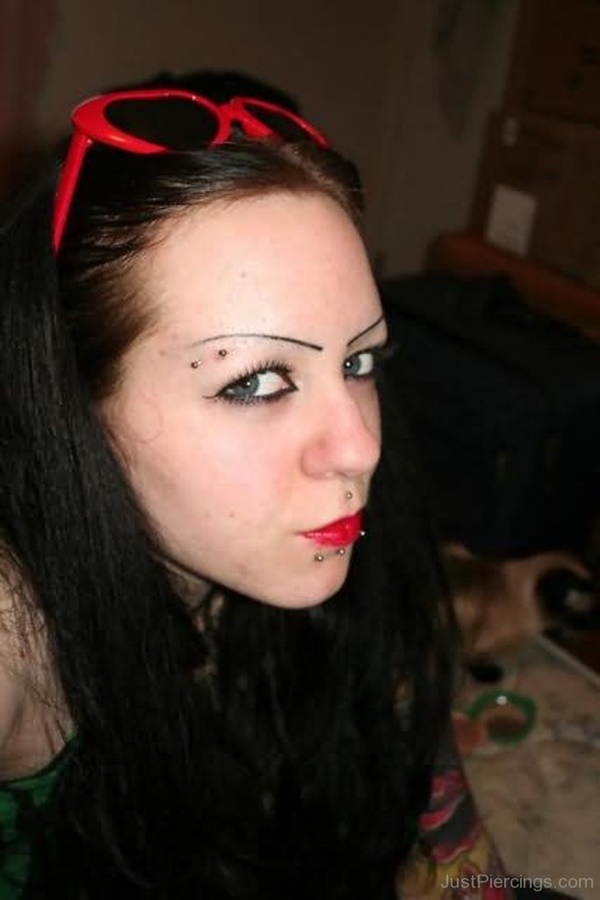This image features a young Caucasian woman with a fair complexion, centered slightly to the left and looking directly at the camera. She has long, dark black hair pulled back and held by a pair of red sunglasses perched atop her head. Her eyebrows are notably plucked or trimmed to narrow lines and are distinctly painted or drawn. Her blue or blue-green eyes are accentuated with black eyeliner and mascara. She has several piercings: two on her right eyebrow, a stud in the philtrum (the area between her nose and upper lip), and three stud piercings below her lower lip. She wears bright red lipstick that prominently highlights her lips. The visible portion of her outfit includes a green tank top, and on her left arm, there is a tattoo. The background is dark and blurry, possibly showing indistinct tubs or furniture, indicating an indoor setting. The overall impression is that she is in a good mood, posing confidently for the photo.